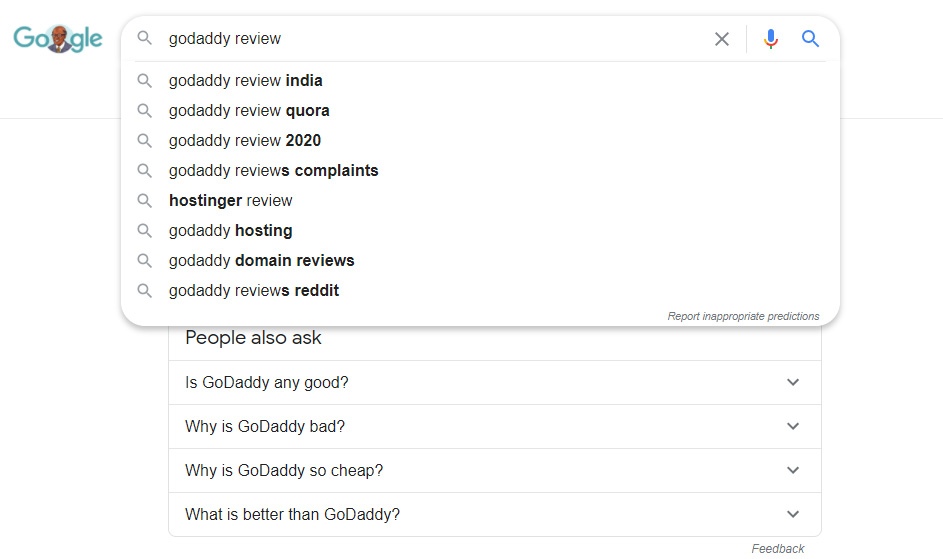The image features a clean, white background. In the upper left corner, there is the website’s logo, which incorporates a small circular image of an African-American man representing the 'O' in the word 'Google'. At the top of the image, a Google search bar reads "Go Daddy Review" in gray text. To the right of the search bar, there are two familiar Google icons: a microphone and a blue magnifying glass.

Below the search bar, a dropdown list appears with several related search suggestions. These suggestions include: "Go Daddy Review India" (with 'India' in bold), "Go Daddy Review Quora", "Go Daddy Review 2020", "Go Daddy Reviews Complaints", "Hostinger Review", "Go Daddy Hosting", "Go Daddy Domain Reviews" (with this entire phrase in bold black text), and "Go Daddy Reviews Reddit". In the lower right corner of the dropdown, small gray text reads "Report inappropriate predictions".

Beneath the dropdown, the phrase "People also ask" is displayed in large, gray text.